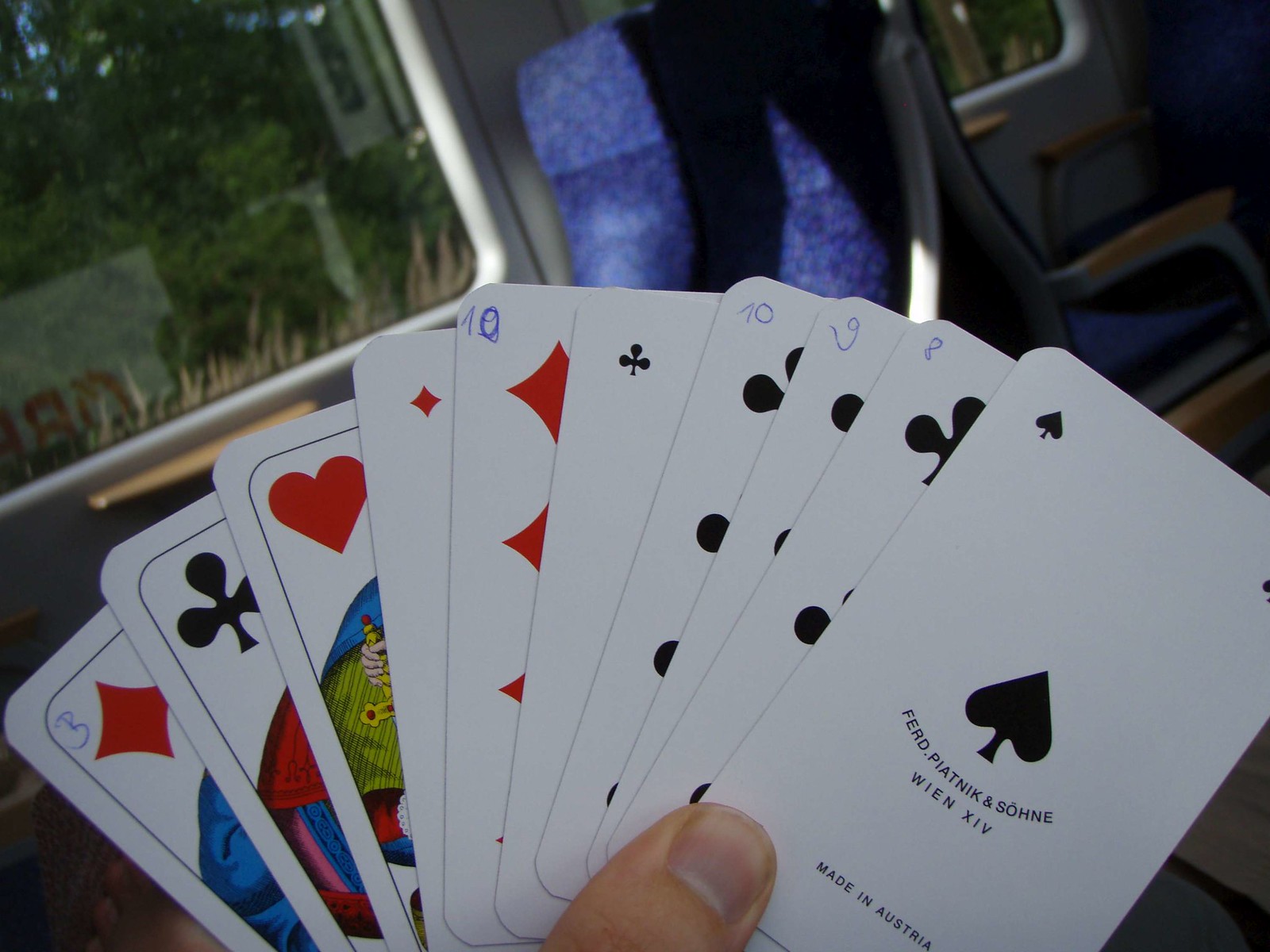A person is shown holding a set of intricately designed cards, fanned out in their hand. These cards are not from a typical deck; they appear to be vintage or custom-made. Prominently displayed among the cards is an Ace of Clubs, which features ornate writing beneath the club symbol: "Pharaoh, Platnick, and Sohne," along with "Wien XIV" and "Made in Austria."

Adjacent to the Ace are three more club cards, labeled with what seems to be handwritten numbers: 8, 9, and 10. Following these is another card showcasing a small club symbol. Next in the hand are two diamond cards, one marked with a handwritten 10 and the other displaying a small diamond.

Further along is a heart card, partially obscured but likely adorned with a picture, possibly a queen. Another club card follows, featuring a large club symbol and another vivid illustration. The final card in the hand is a diamond, marked with the handwritten number 3, accompanied by a faint, barely visible drawing.

The collection of cards is vividly colorful, incorporating hues of red, black, purple, white, blue, and green, highlighting the detailed illustrations and handwritten elements on each card.